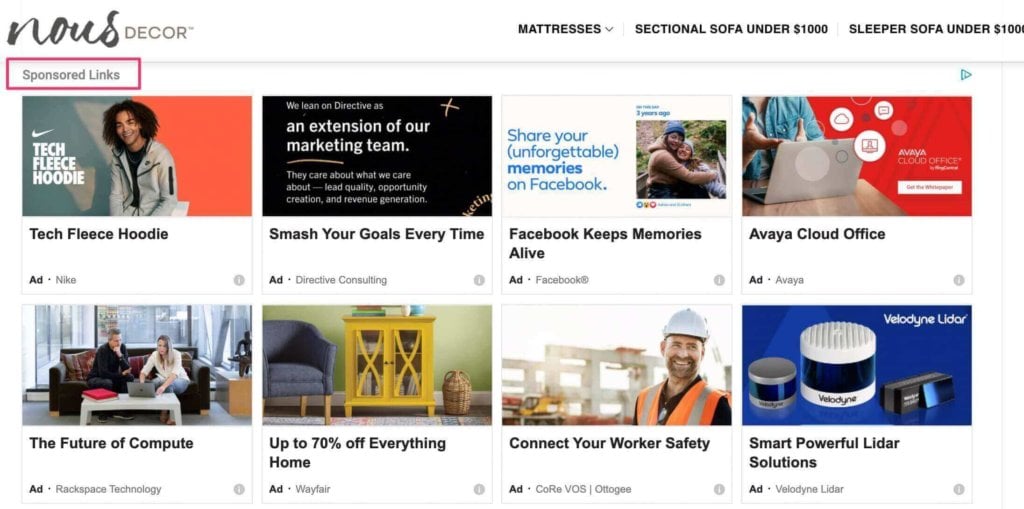This image is a screenshot from a website named "NUSH Décor." The word "NUSH" is written in a stylish cursive font, all in lowercase letters, while "DÉCOR" is displayed in bold, uppercase black letters. Positioned at the top of the page are several dropdown menus featuring options such as "mattresses," "sectional sofa under $1,000," and "sleeper sofa under $1,000." 

A prominent red rectangle highlights a section labeled "sponsored links," drawing attention to this area. In this section, multiple advertisements are displayed. Among them, a Nike ad promotes a "tech fleece hoodie." Another ad encourages individuals to "smash your goals every time" with the help of Directive as an extension of their marketing team. Additionally, there is an ad about Facebook, suggesting users "share your unforgettable memories" to keep them alive. The final ad in the top row is for "IEA cloud office."

Similarly, the bottom row of the screenshot houses an additional four ads, maintaining the overall layout and theme of the webpage.